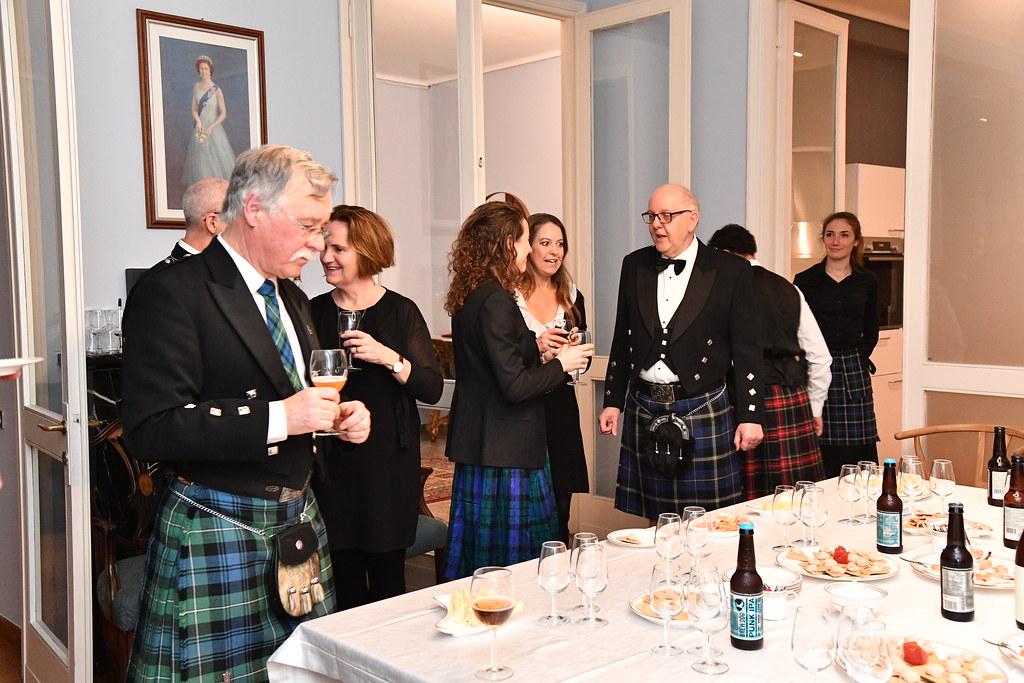In a well-lit room with light blue walls, eight people gather, all adorned in traditional Scottish attire featuring kilts and coordinated accessories. The scene appears to be a sophisticated reception or social event. Toward the left, an open door with white borders reveals a smaller adjacent room containing a white refrigerator. Above, a framed portrait of Queen Elizabeth graces the blue wall, and nearby, another door with glass panes stands partially open. 

At the center, a man with shaggy gray hair, sporting a black jacket, white button-up shirt, blue and green striped tie, and a matching kilt with a fanny pack, raises a nearly empty wine glass. Directly in front of him, a short-haired woman in a long black shirt and black pants adds to the crowd's charm. Behind her, a woman with brown upper-back-length hair, dressed in a black sports coat and a blue and green kilt, holds a wine glass.

To their right, another woman with hair falling just below her shoulders stands elegantly in a black dress accented with white ruffles at the neck. Further right, an older gentleman with balding hair and glasses, attired in a white shirt, black bow tie, black jacket, and a blue and black kilt, stands with his arms by his sides.

A woman to his left, seen only from the back, wears a black shirt with white sleeves and a red and black kilt. On the far right, a young girl with short hair, dressed in a long black shirt and a blue and black kilt, stands in an open doorway, looking to the right.

In the bottom right corner of the image, a large white table brimming with empty wine glasses, bottles resembling beer, and various dishes of food and snacks adds to the festive atmosphere. The ambiance suggests a gathering filled with conversation, cultural pride, and shared company, all under the gaze of a regal portrait.